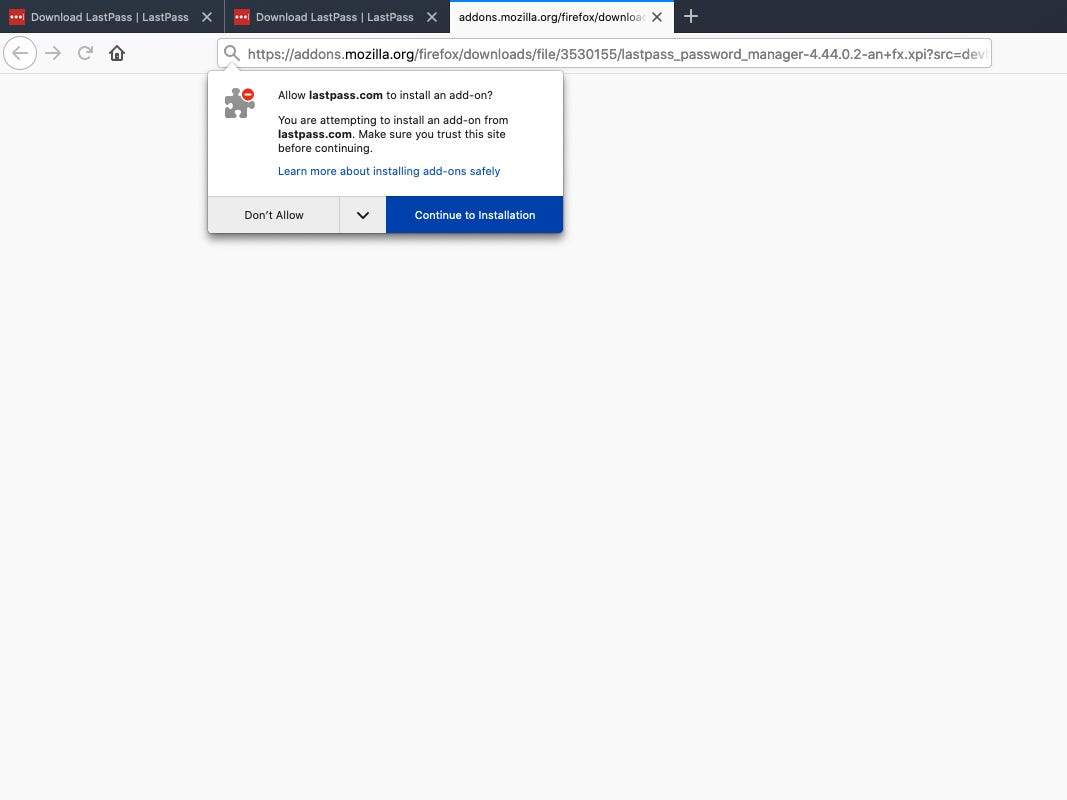A screenshot captures a web browser window with three open tabs displayed in the Firefox browser. The highlighted tab shows the URL: "addons.mozilla.org/Firefox/downloads/file" and indicates it's from the Mozilla website. The browser interface includes a pop-up message originating from a small magnifying glass icon. The message reads: "Allow lastpass.com to install an add-on. You are attempting to install an add-on from lastpass.com. Make sure you trust this site before continuing." Below the message, blue text offers a link to "Learn more about installing add-ons safely." Two buttons are available; the left one, marked "Don't Allow" with a downward arrow, and the right one, a blue button that states "Continue to Installation." The two adjacent browser tabs also have the title "Download LastPass" with a red icon beside each. The main web page displayed in the screenshot is entirely blank.